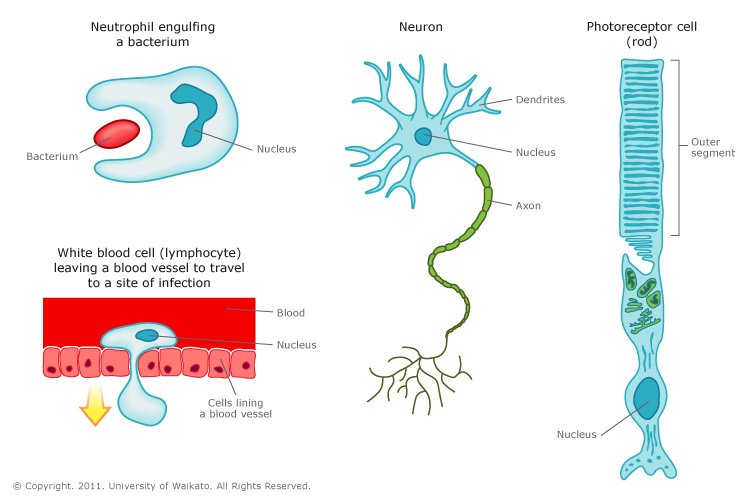The image displays four detailed biology illustrations against a white background. In the top left corner, the illustration depicts a neutrophil engulfing a bacterium, labeled as such. The visual shows a large blue nucleus inside a bigger blue shape, surrounding a smaller red circle representing the bacterium. Arrows point to these parts, clearly labeling the bacterium and the nucleus. Below this, on the lower left, there's an illustration of a white blood cell, specifically a lymphocyte, leaving a blood vessel to travel to the site of infection. It features a red rectangular area labeled "blood," from which a blue shape with a nucleus (colored blue) appears to seep out. Scattered red blobs next to the blue shape are labeled as cells lining the blood vessel, with a yellow arrow indicating the direction of movement. The top right illustration shows a neuron, with clear labels for its dendrites, nucleus, and axon. The dendrites branch out from the neuron like tree limbs, while the axon extends as a green tail-like structure. Lastly, the bottom right image illustrates a photoreceptor cell rod. This long blue structure includes a segmented part labeled "outer segment" and a circular nucleus at the lower end. Each element is meticulously labeled, offering a comprehensive visual guide to these biological components.